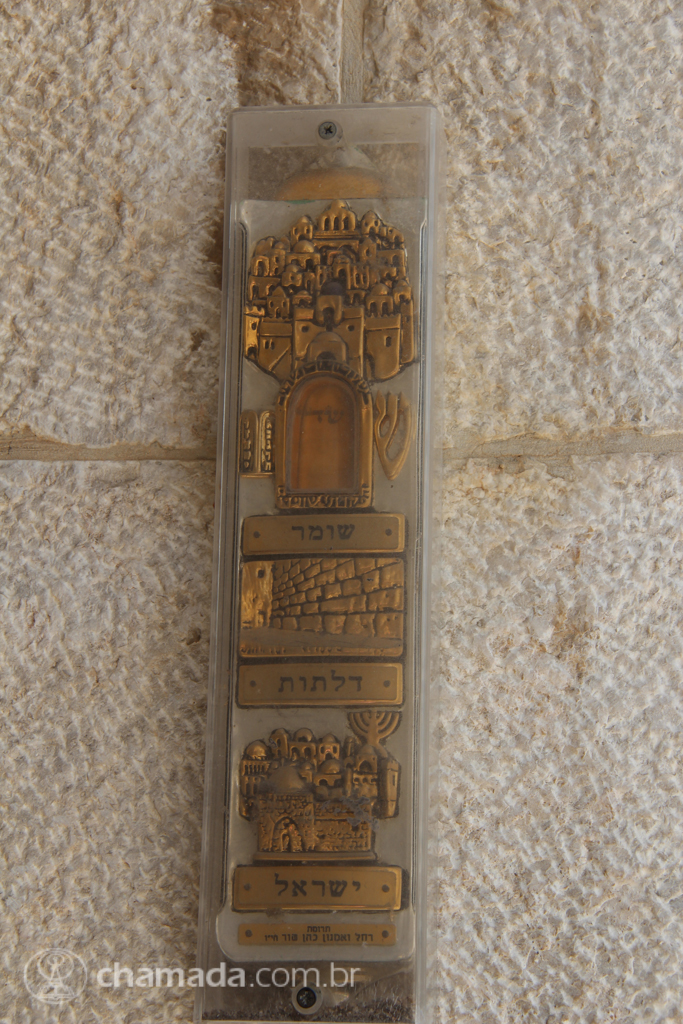The photograph captures a textured, white brick wall with a small, thin plastic plaque screwed into it. The plaque features intricate engravings made out of copper, depicting a cityscape, a large door, a brick wall, and another city from top to bottom. In the bottom left corner, bold white text reads "Shemada," while next to it in grey font is "chamata.com.br."